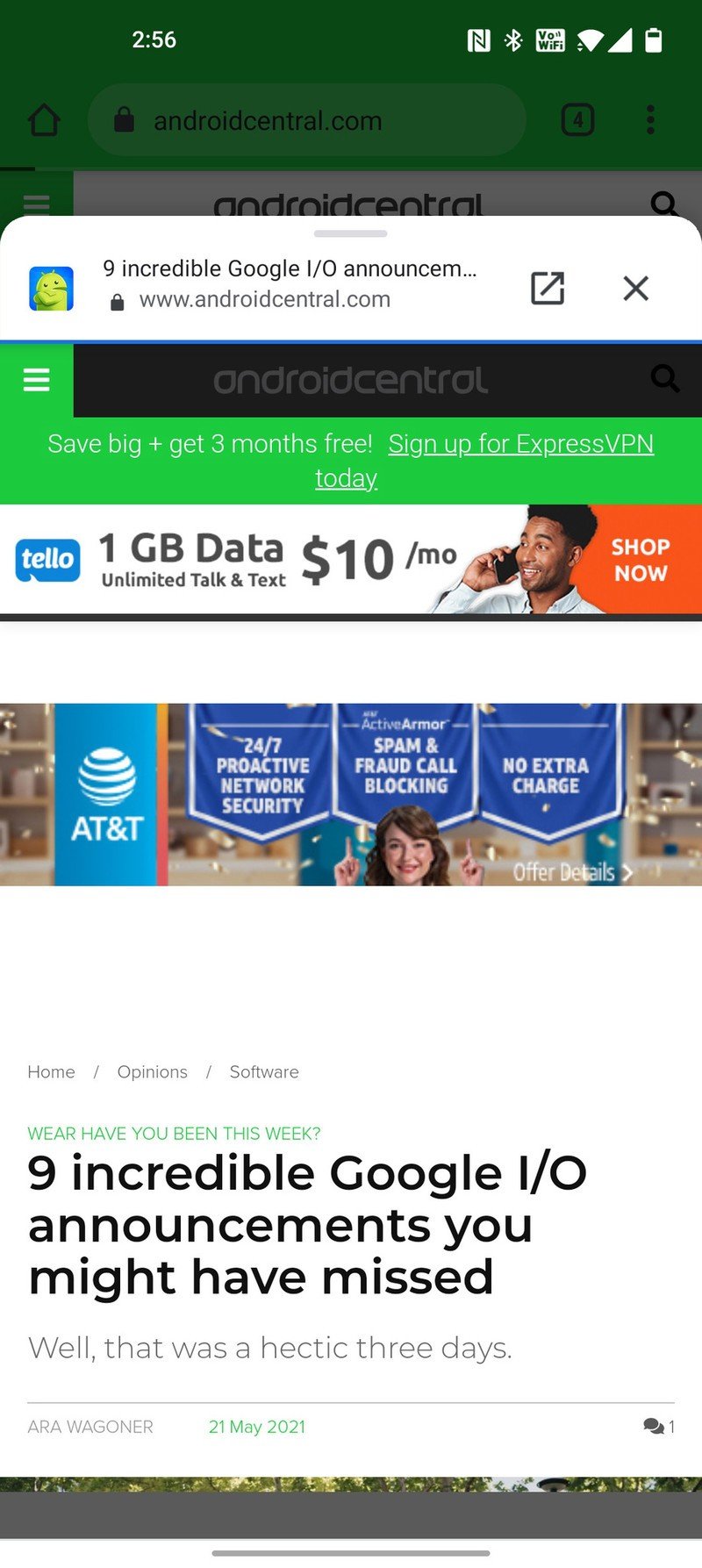The image is a screenshot of a cell phone displaying the androidcentral.com website. In the top right corner of the phone's screen, the battery icon indicates approximately three-quarters charge. Adjacent to the battery icon are symbols representing full bars for cellular connection and Wi-Fi signal strength. There is also a white square with words, a Bluetooth icon, and an 'N' on a white background.

On the upper left-hand side of the screen, the number '256' is displayed. As you move down the webpage, the Android Central logo is visible against a subdued gray background.

The primary content of the webpage includes a prominent tab that reads, "9 Incredible Google I/O Announcements," with an "X" close button in the upper right corner of this tab. Beneath it, there's a green drop-down menu offering a promotion: "Save big plus get three months free – Sign up for ExpressVPN today."

Further down, an advertisement banner for Tello features on a white background, offering "1 GB data, unlimited talk and text for $10 a month" along with a "Shop Now" button.

Another advertisement below it showcases AT&T, with the AT&T spokesperson pointing at banners highlighting features such as "24/7 proactive network security," "Spam and fraudulent call blocking," and "No extra charge."

Lastly, the article headline "9 Incredible Google I/O Announcements You Might Have Missed" is prominently displayed towards the bottom of the screen.